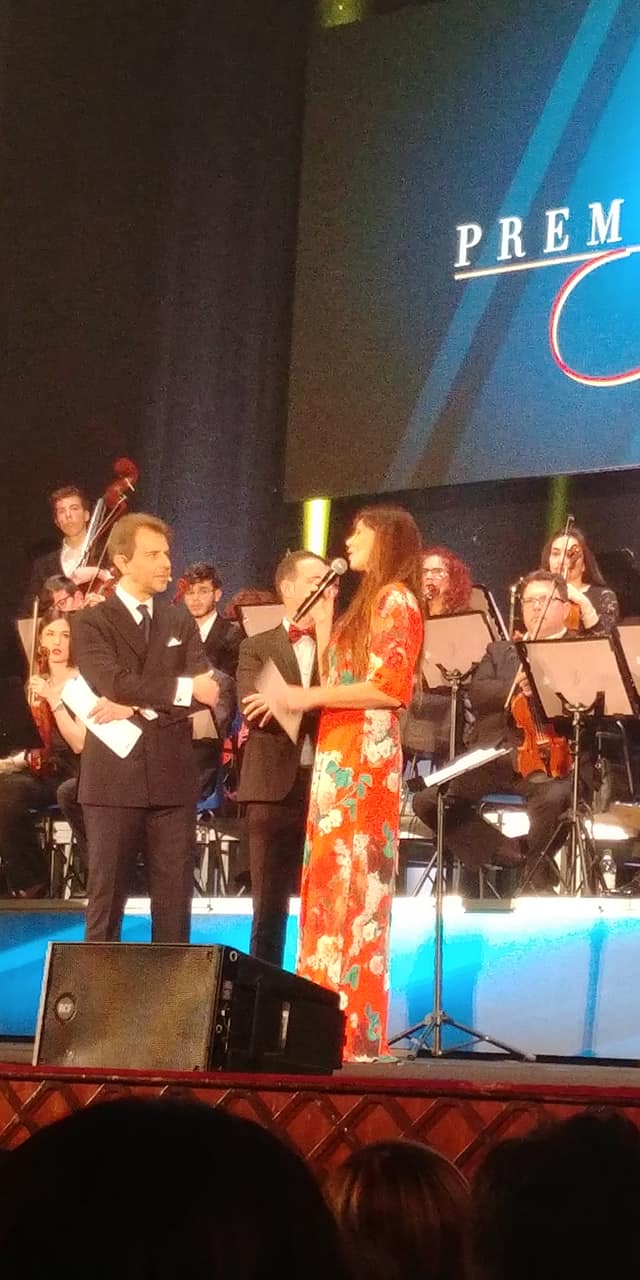On a tall, narrow stage, a woman in a vibrant floor-length orange dress adorned with white floral patterns stands holding a microphone with her right hand, and a piece of paper or an envelope with her left. She faces a man in a dark suit, who stands with his arms crossed, holding a white sheet of paper. The man's gaze is fixed on the woman as she speaks into the microphone. Behind them, an orchestra of about half a dozen musicians, including violinists and a bassist, sit poised with their instruments and sheet music stands, though they are not currently playing. The backdrop features curtains and a partially visible banner with the letters "PREM." At the edge of the stage, there's an amplifier lying on its side, and the lower part of the image shows the heads of audience members watching the scene.